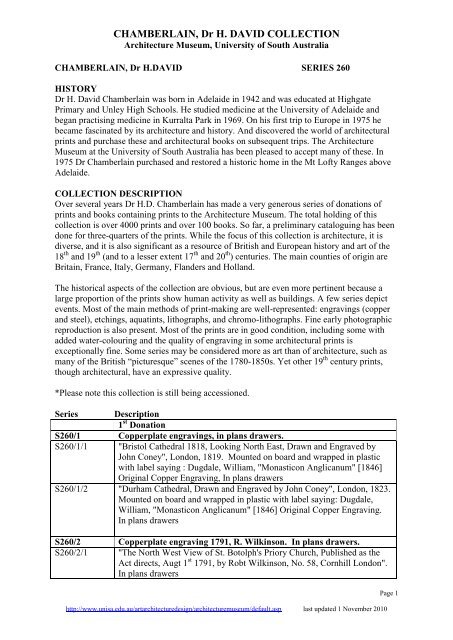The image is a text document from the University of South Australia's Architecture Museum, detailing the Chamberlain, Dr. H. David Collection, Series 260. The document features a white background with black text and includes multiple sections. At the top, it introduces Dr. H. David Chamberlain, born in Adelaide in 1942, educated at Highgate Primary and Unley High Schools, and trained in medicine at the University of Adelaide. The history section details his journey from practicing medicine in Caralta Park starting in 1969 to developing a fascination with European architecture during his travels in 1975, ultimately resulting in his restoration of historic homes. The collection description provides an overview of the items he donated, which includes prints and books that are significant to architectural history. At the bottom of the document, there is a small table summarizing these donations, along with a blue hyperlink.